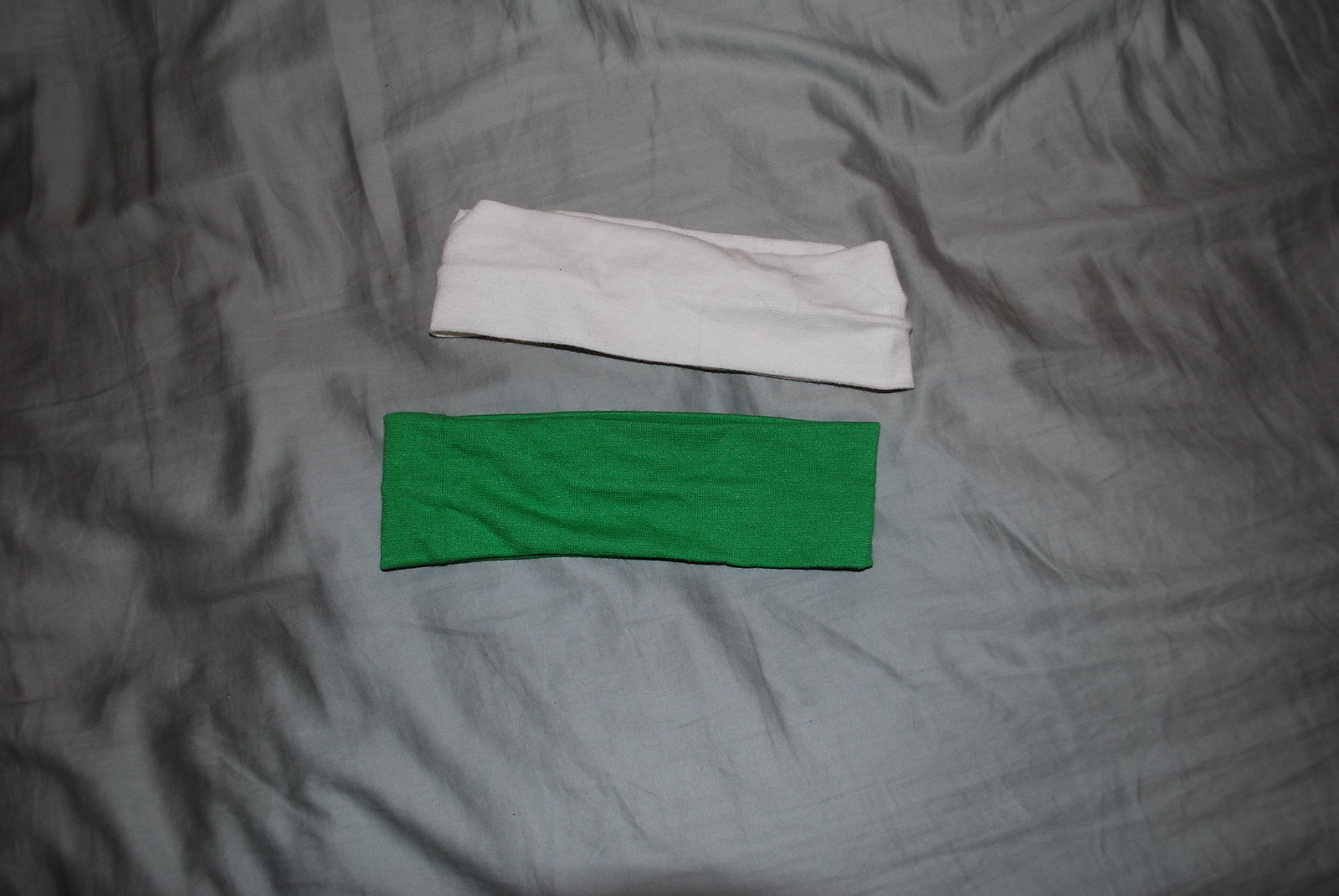The photograph captures a slightly wrinkled gray sheet, likely made of satin, covering a surface that could be a bed. In the center of the sheet lie two rectangular strips of felt-like cloth, one white and one dark green, with the white piece on top. Both pieces of felt are noticeably wrinkled and somewhat bunched, creating an imperfect, slightly disordered appearance. The gray sheet itself features larger folds and wrinkles concentrated in the upper and left portions of the image, while the lower right appears smoother. A prominent light source illuminates the center of the photograph, emphasizing the textures and folds of the fabrics.